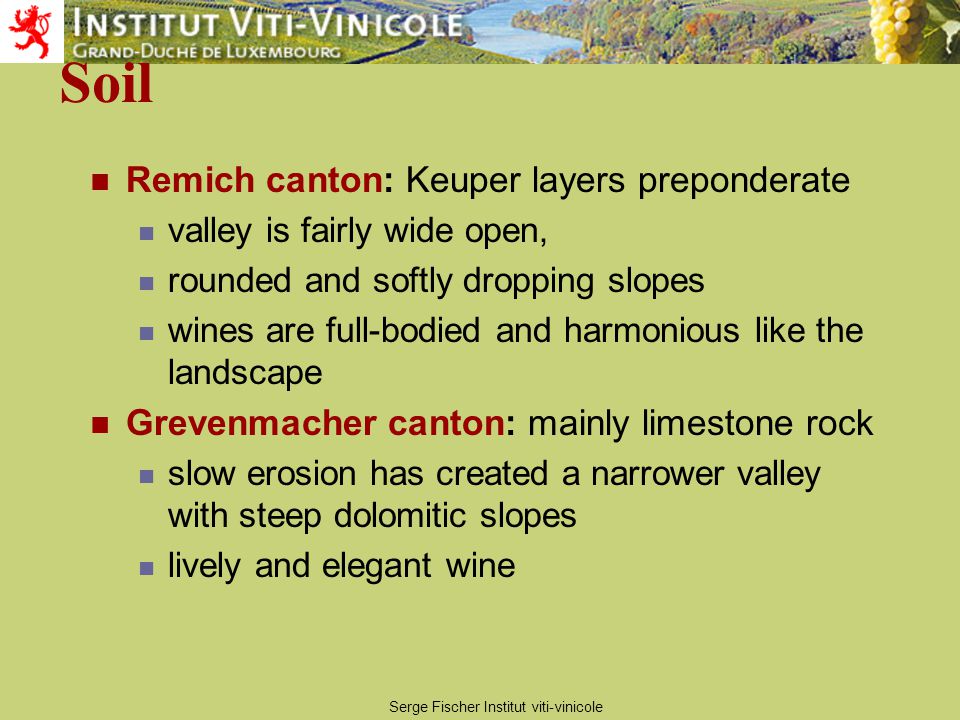The poster, set against an earthy green background, prominently features the name of an institute at the top: "Institut Viticole Grand Duché de Luxembourg." On the upper left corner, there's a red lion logo facing left, emblematic of the institute. Adjacent to the logo, the text "Institut Viticole" appears, followed by "Grand Duché de Luxembourg." Centrally placed below, a landscape image depicts a verdant valley with a meandering blue river, trees, and a hint of yellow that resembles corn. Beneath this, the main title "Soil" is presented in striking red font.

The poster details two primary regions: 

1. **Remich Canton**: 
   - Kimmeridgian layers predominate.
   - Valley is fairly wide open.
   - Rounded, softly dipping slopes.
   - Vines are full-bodied and harmonious, mirroring the lighter landscape.

2. **Grevenmacher Canton**:
   - Mainly limestone rock.
   - Slow erosion has formed a narrow valley with steep dolomitic slopes.
   - Vines are lively and elegant.

Each section is marked by red bullet points, with detailed descriptions in black text.